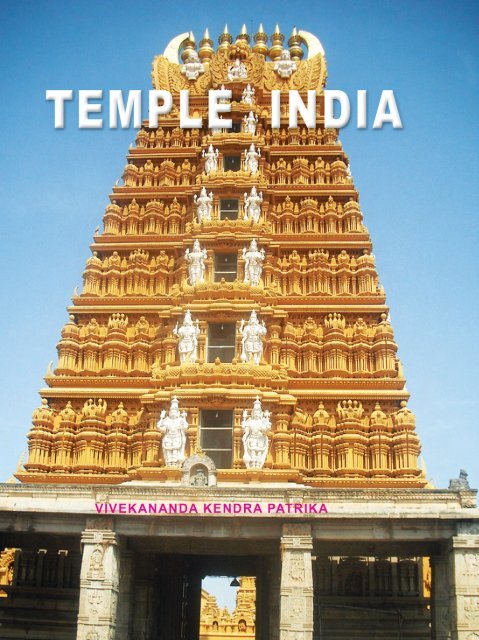The image features a magnificently ornate temple in India, prominently showcasing a combination of golden and white hues. The temple structure is grand and towering, comprising seven distinct levels, each adorned with intricate details. Flanking each of the windows on these levels are two white statues—one on each side—resulting in a total of 14 statues that enhance the temple's architectural elegance. The design intricacy signifies the immense effort and craftsmanship that went into constructing this edifice.

The lower part of the temple, crafted from a dark gray stone, includes an entranceway leading to a courtyard, where similar orange-hued buildings can be glimpsed. The entrance frame features purple writing, "Viva Kannada Kendra Patrika." The architectural form tapers into a triangular shape, although the very top of the temple is cut off in the photograph. Overlaying the top section of the image is the text "Temple India" in striking blue and white lettering. The background of the image is characterized by a bright, cloudless blue sky, adding to the serene and majestic atmosphere of the scene.